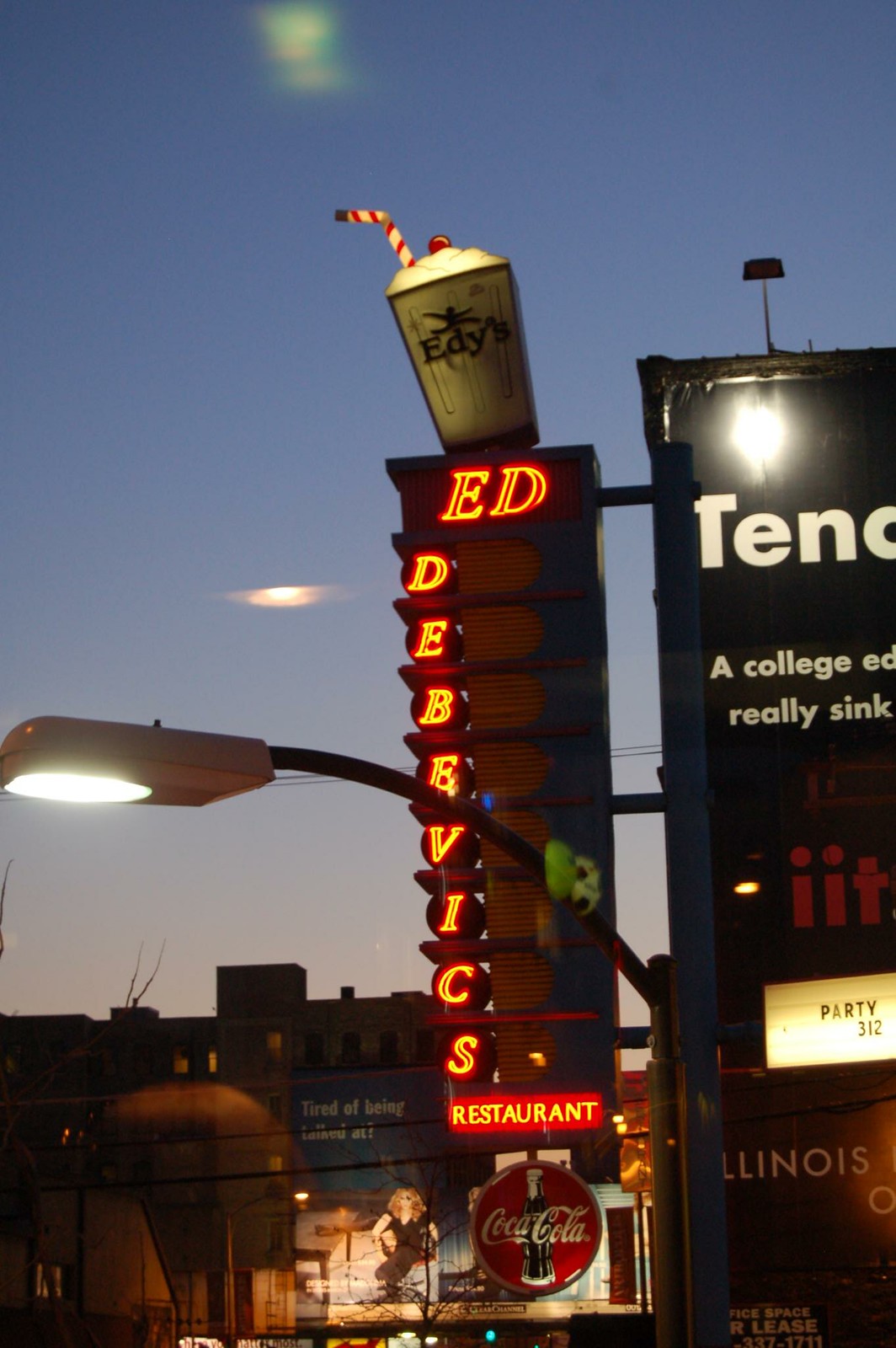The image depicts a vibrant street scene at twilight, featuring a large, eye-catching neon sign attached to a building on a busy street. The sign, illuminated against the dusky sky, prominently displays a giant milkshake container adorned with a red and white striped bendy straw, whipped cream, and a cherry, with the word "EDIS" written across it. Below this, vertically stacked neon letters spell out "Ed DeBevick's Restaurant," with "Restaurant" lit by regular illumination instead of neon. Below this main sign, a classic circular Coca-Cola logo in red and white stands out. Directly beneath the Coca-Cola sign, an illuminated box reads "Party 312," followed by another sign that says "Illinois." A nearby billboard partially visible to the right has obscured text. The bright streetlamp in the foreground adds to the nighttime ambiance, contrasting with the clear, blue-tinted twilight sky devoid of clouds and people.